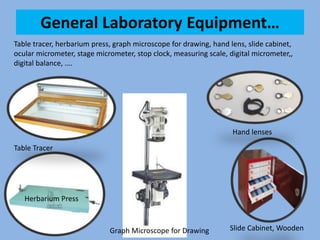This is a small, computerized infographic with a blue background, likely clipped from a web page, measuring approximately one and a half by one and a half inches. At the top, a light blue rectangle features the black text “General Laboratory Equipment,” followed by an ellipsis. Below this heading, there is a list that includes items such as a table tracer, herbarium press, graph microscope for drawing, hand lenses, slide cabinet, ocular micrometer, stage micrometer, stop clock, measuring scale, digital micrometer, and digital balance. 

The infographic showcases images of four specific devices in oval frames with black outlines. On the left side, the top oval contains an image of a table tracer, while the bottom oval shows an herbarium press. On the right, the top oval depicts hand lenses, and the bottom oval displays a wooden slide cabinet. Centrally, a white rectangular section highlights a graph microscope for drawing, providing a detailed representation of the equipment. The meticulous layout and labeled visuals clearly identify the various pieces of laboratory equipment presented.